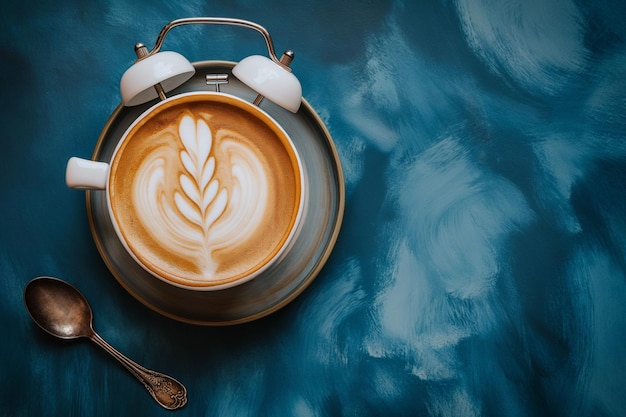The image features a stylish coffee scene set against a deep blue, painterly background scattered with white smudges and brush strokes, particularly heavy on the right side. In the foreground, a white coffee cup sits slightly off-center on a silver saucer-like tray. The coffee, a light tan latte, showcases an intricate fern leaf design in its foam, indicating skilled barista craftsmanship. Notably, the cup is whimsically topped with the twin bells of an alarm clock, merging the everyday allure of a morning coffee with the jarring familiarity of an alarm. A small coffee spoon resides just to the bottom left of the cup, completing this serene yet artistic portrayal of a coffee break moment.